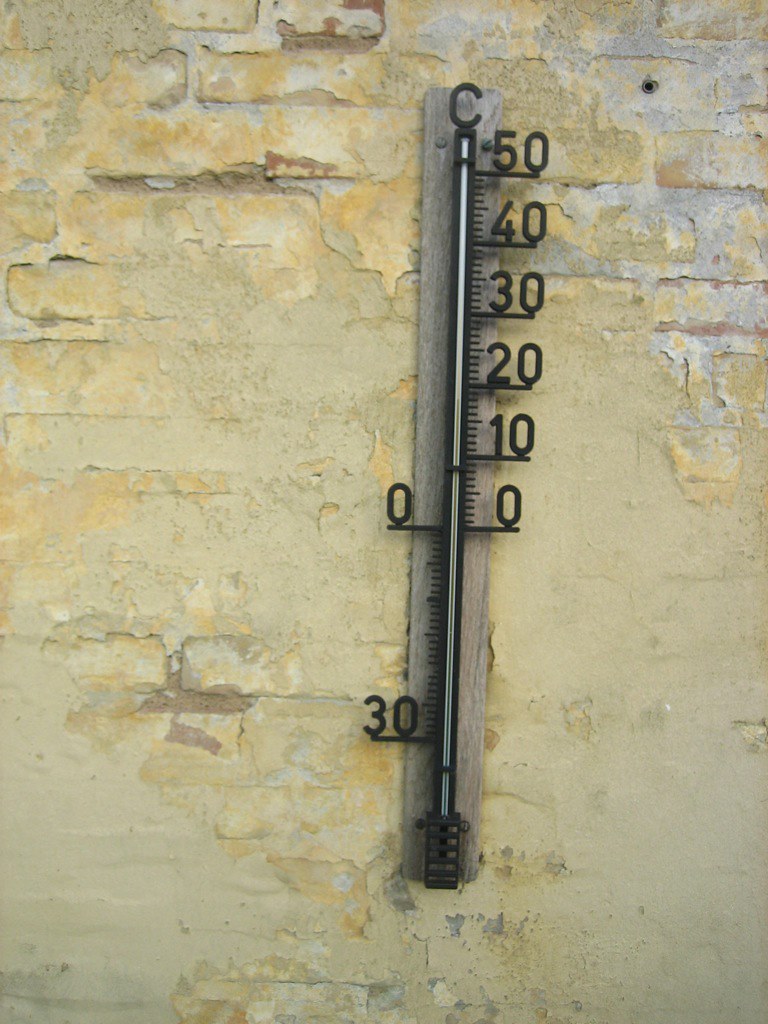The image showcases an aged brick wall with a distressed, worn appearance. The bricks have a rich, gold hue intermixed with subtle white and cream accents, hinting at years of wear and weathering. Mounted on the wall is an antique thermometer, crafted from a long wooden plank, possibly a 2x1 or 2x4, and approximately three feet in length. The thermometer's wooden base exudes an old-world charm, complementing the rustic backdrop. At the top, an iron line forms a "C," denoting Celsius. The thermometer is marked with descending numbers: 50, 40, 30, 20, 10, and finally zero at the center. On the left side, the scale continues downward, marking degrees below zero, reaching up to -30 degrees Celsius.